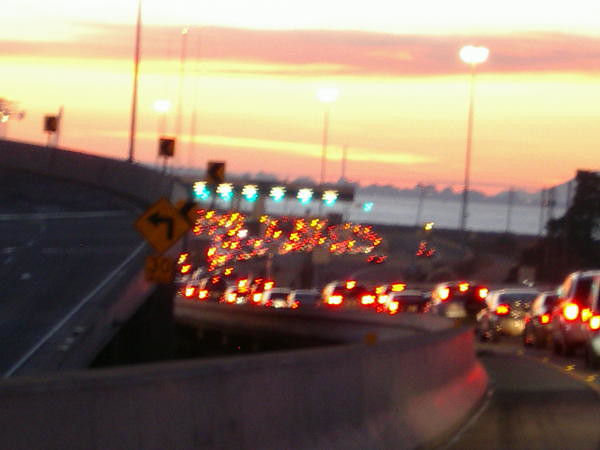The image depicts a bustling highway scene during dusk, characterized by heavy traffic with numerous cars emitting red taillights. The vehicles are merging from an overpass onto a toll road. The sky is a captivating gradient of bright pink, yellow, and orange hues, indicative of a sunset that has almost fully set. The scene features a clutter of cars navigating a curve, guided by several yellow traffic signs with black arrows pointing left, indicating the turn should be taken at 30 mph. In the background, there's a silhouetted skyline of tall buildings and a body of water, possibly an ocean or bay, adding depth to the image. The streetlights are turned on, illuminating the highway with their artificial glow, accentuating the busy and slightly blurred nature of the scene.